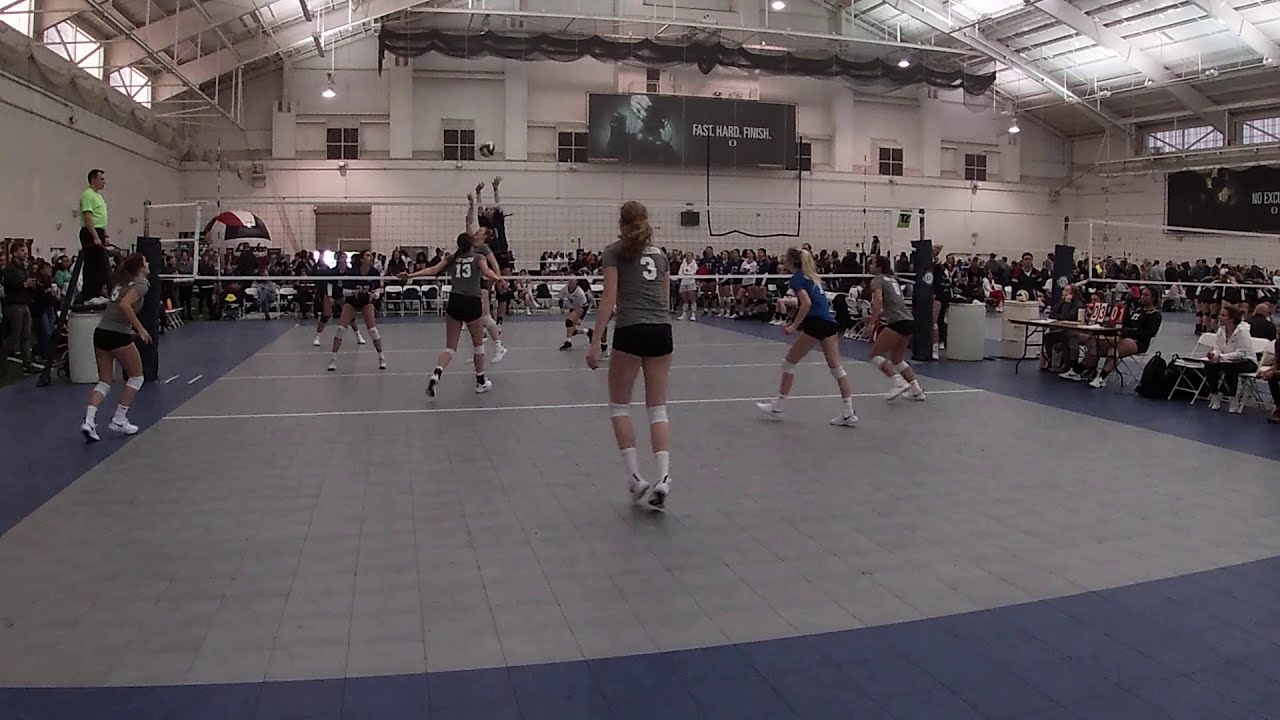The image captures a vibrant scene of an indoor gymnasium during a volleyball match, viewed from the short end of the volleyball court. The gymnasium's white and blue-floored court is lined with green tiled walkways. Five players, wearing gray or blue t-shirts with white numbers and black shorts, are positioned near the net, with their backs facing the camera, indicating a game in progress. Positioned on a platform near the left side of the net, a referee in a neon yellow or green shirt oversees the match. The gymnasium's high, gray metallic ceiling features skylights and multiple lights, illuminating the entire space.

Surrounding the court, spectators fill several rows of folding chairs, creating a lively atmosphere. Numerous onlookers suggest a well-attended event, possibly featuring multiple teams and schools. An encouraging banner with the words "Fast Hard Finish" and accompanying graphics decorates one of the walls. The presence of active scorekeepers and the structured setup indicates a formal match, though it could also be a warm-up session. Overall, the image details a bustling volleyball tournament, capturing the energy and enthusiasm of both players and spectators.